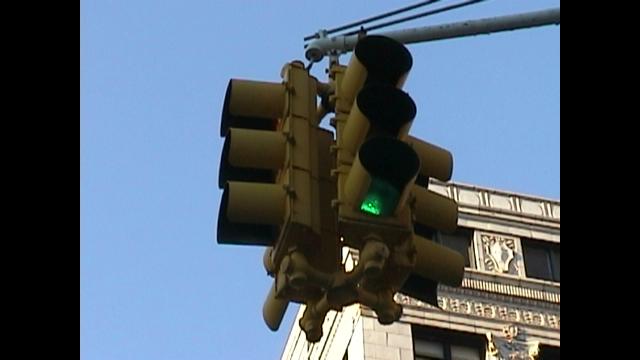This photograph captures a cluster of four-way, vintage-style streetlights hanging from a horizontal pole at an intersection. The lights, in yellow metal with cylindrical tubes shielding each bulb, aim outward in four directions. The visible front light is green, illuminated in the bottom cylinder. The streetlights are mounted on a steel-gray beam that enters the frame from the top right. Set against a clear, light blue sky, the scene includes a tall, ornate gray brick building in the bottom right corner, adorned with decorative cornices, relief carvings, and open windows. The image is framed with black bars on the left and right sides, focusing attention on the central composition.